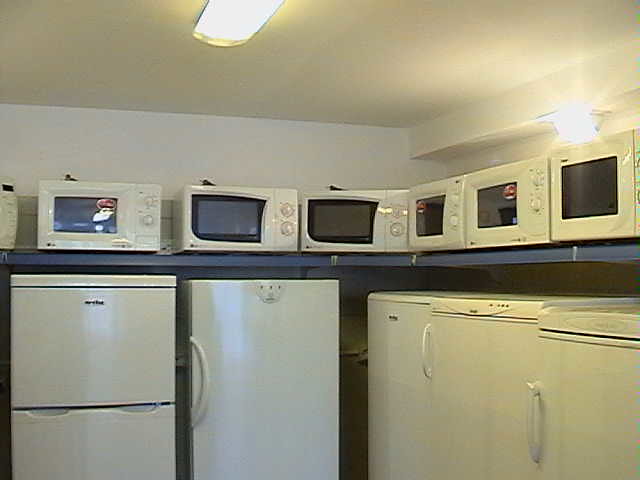This image captures the corner of a white-walled appliance store, brightly illuminated by two fluorescent lights—one on the ceiling and one on the top right of the frame. Dominating the corner is a blue painted wooden shelf positioned at shoulder level. Resting on this shelf are six white microwave ovens, each model slightly differing from the others, particularly in their control panels. Below the shelf, on the floor, are five European-style upright refrigerators, easily recognizable by their left-sided handles and relatively shorter height, extending just below shoulder level. The fridges share a uniform white color, consistent with the microwaves above. The scene suggests an organized display of appliances, perhaps for sale, highlighting the comparative consistency in design while offering subtle variations in functionality. The overall lighting casts some reflections and shadows, adding depth and hints of morning light to the setting.